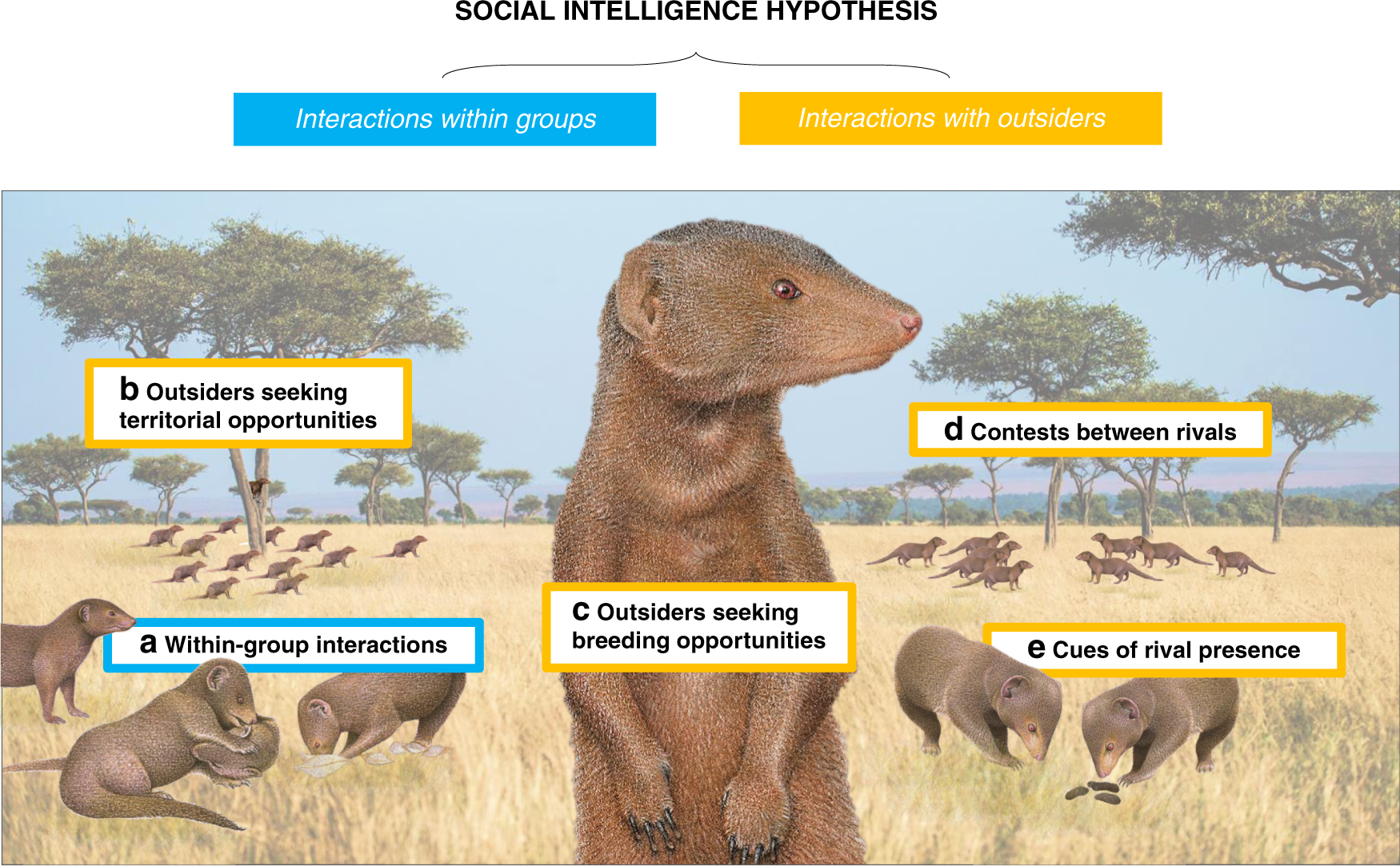The image is a detailed infographic styled with colorful and lifelike digital drawings, likely designed for educational purposes. The main heading at the top reads "Social Intelligence Hypothesis" against a white background. The content is divided into two main sections: "Interactions Within Groups" encased in a blue box, and "Interactions With Outsiders" in a yellow box.

The scene depicted is reminiscent of the African Savannah, featuring a landscape with golden grass, large trees, a blue sky, and distant hills. Among the scenery, brown mongoose-like creatures with fuzzy fur, pointy faces, pink noses, black claws, and brownish eyes are engaged in different activities, each labeled with specific interactions highlighted by various colored boxes:

- **A: Within Group Interactions** (blue box) shows the animals engaging in social activities within their group.
- **B: Outsiders Seeking Territorial Opportunities** (yellow box) illustrates the animals running, symbolizing the quest for new territories.
- **C: Outsiders Seeking Breeding Opportunities** (yellow box) features a single animal standing in the center, looking sideways, emphasizing individual pursuits for mating.
- **D: Contests Between Rivals** (yellow box) depicts groups of animals facing off against each other, showcasing competitive behavior.
- **E: Cues of Rival Presence** (yellow box) presents two animals intently observing something on the ground, possibly sniffing for signs of competitors.

The illustration captures the essence of social interactions among these creatures, both within their groups and with outsiders, aligning with the concept of the Social Intelligence Hypothesis.